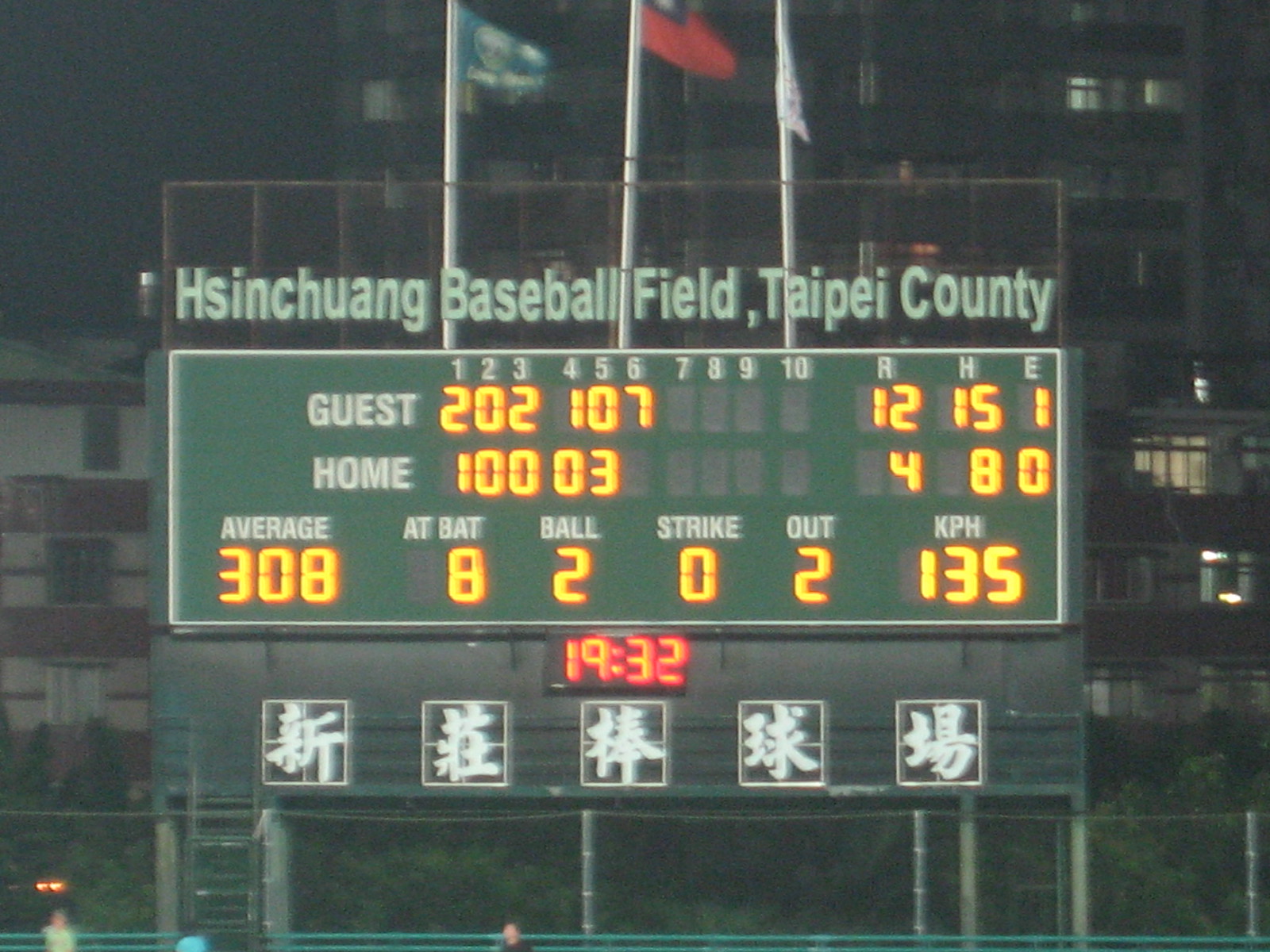The image portrays a photograph of a baseball scoreboard at the Hsinchuang Baseball Field in Taipei County. The scene is set at night, indicated by illuminated buildings and a dim background. The scoreboard prominently displays the fields "Guest" and "Home" with scores for each inning listed from 1 through 10. To the far right of the inning counts, it notes R (runs), H (hits), and E (errors) with guest leading 12 to 4 by the end of the sixth inning. In yellow, detailed stats such as an average of 308, 8 at-bats, 2 balls, 0 strikes, 2 outs, and a pitch speed of 135 KPH are shown. The time, displayed in red lights, reads 19:32, and immediately below, five Chinese characters can be seen. The board is flanked by a chain-link fence and some people, hinting at the game’s ongoing nature. The overall atmosphere is reflective of an engaged community gathered for a local baseball game in a Chinese-speaking region.